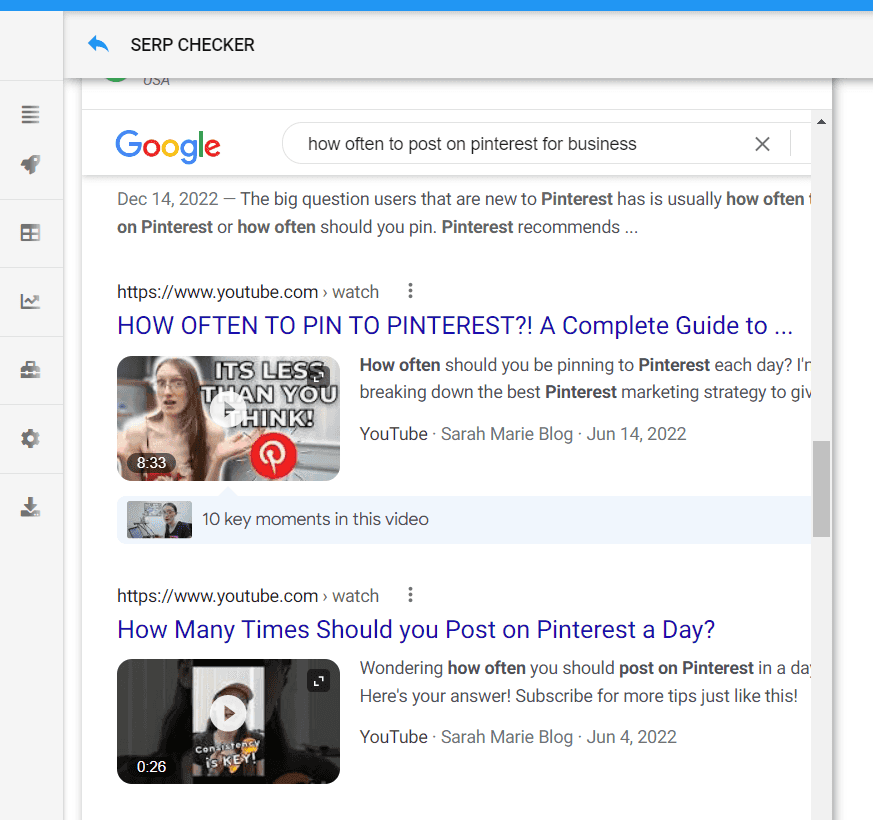A detailed screenshot of a web page is shown, specifically displaying the interface of a SERP Checker tool. The top portion of the image features a gray banner with a blue line forming a thin top border. Within this banner, there is a left-pointing arrow accompanied by the text "SERP Checker," where "SERP" is spelled out in capital letters. 

On the left side of the screenshot, a vertical section houses several icons including a unique hamburger icon with four lines, a rocket, a calendar-like symbol, a graph, an image that resembles a lunchbox, gear cogs, and a download icon.

The central part of the image prominently displays the Google search bar with the query "how often to post on Pinterest for business" typed in. An 'X' icon is present within the search bar, indicating an option to clear the query. Below the search bar, search results are visible, starting with the date "December 14, 2022," followed by a section that addresses common questions from new Pinterest users about posting frequency. Part of the text is cut off, but it reads: "The big questions users that are new to Pinterest have. It's usually how often... on Pinterest or how often should you pin. Pinterest recommends..."

Further down, there are two embedded video results. The first one is titled "How often to pin to Pinterest: A complete guide to..." followed by an ellipsis. The second video description reads: "How many times should you post on Pinterest a day," with both videos originating from YouTube.